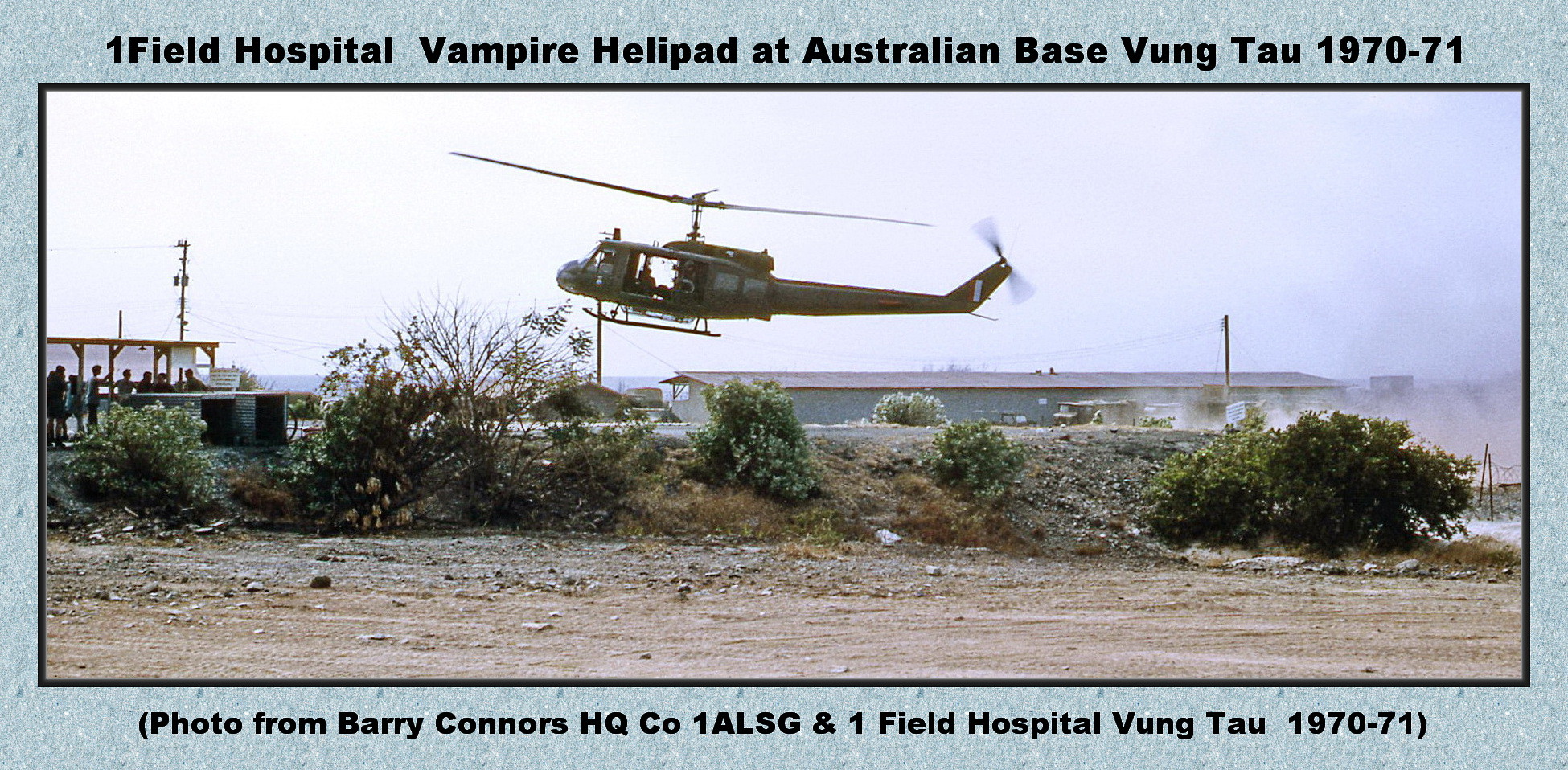This photograph, taken outdoors in the middle of the day during 1970-71 in Vung Tau, Vietnam, is set within a light blue, textured border that features the text, "Onefield Hospital Vampire Helipad at Australian Base, Vung Tau, 1970-71" at the top and "Photo from Barry Connors, HQ Co., 1 ALSG, Onefield Hospital, Vung Tau, 1970-71" at the bottom. Central to the image is a Vietnam-era helicopter, possibly a French model, in the process of landing on a distressingly barren, sandy field that inclines slightly toward the center, where sparse bushes and vegetation are visible. On the left, under a wooden awning with white walls, a few people appear to be standing, while off in the distance to the right, a long cabin can be seen, blending into the modest and utilitarian military base surroundings rendered in a palette of light blue, black, green, brown, tan, and gray hues.